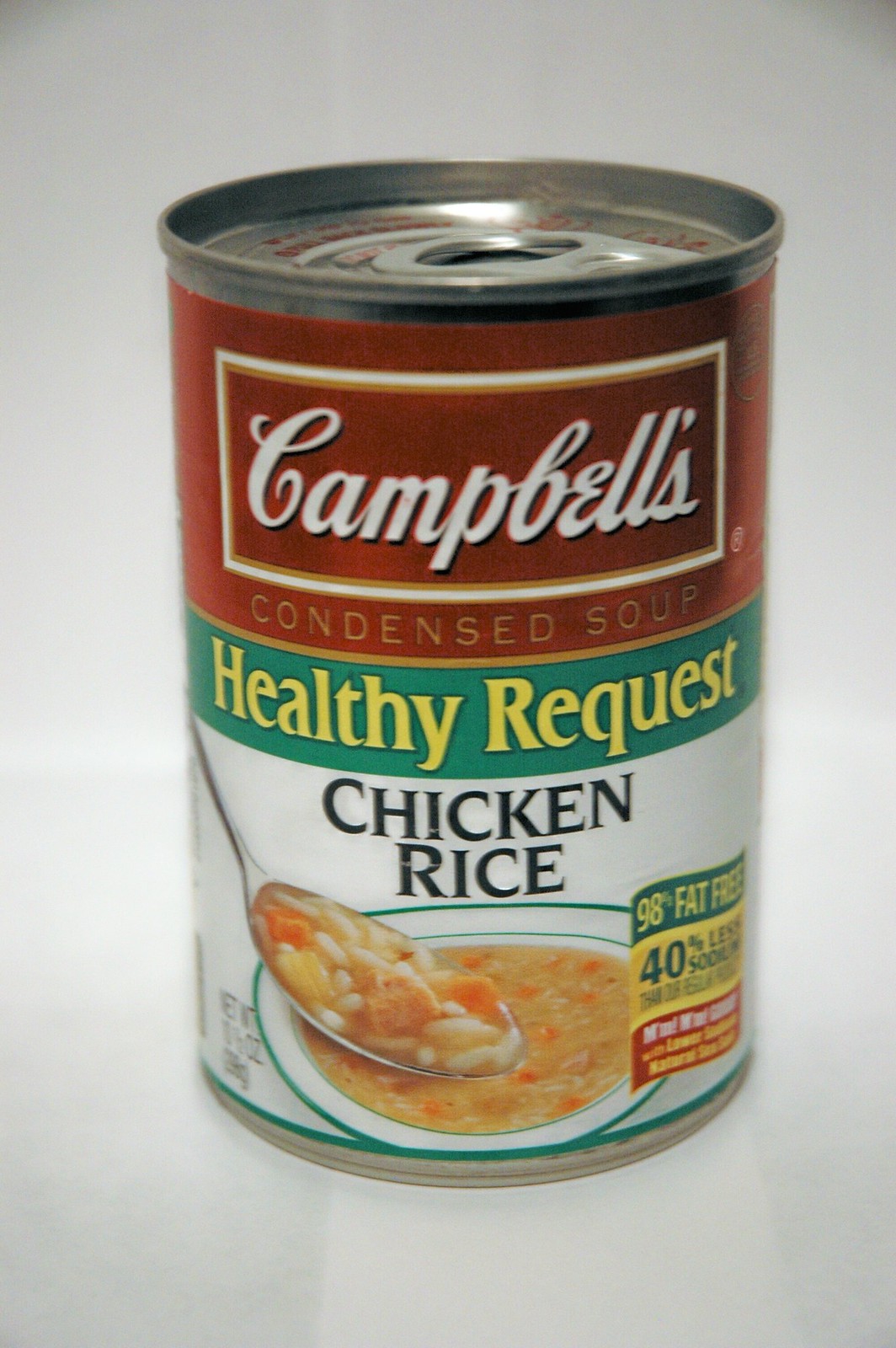A close-up image of a Campbell's Healthy Request Chicken with Rice Soup can, positioned against a clean white background. The can, displaying the traditional Campbell's design, features a pull-tab top viewed at an angle. The "Healthy Request" label is prominently written in yellow on a green background, conveying a sense of healthiness. Beneath the label is a detailed image of a white bowl with green concentric rings, filled with the hearty chicken and rice soup. In the soup, visible chunks of rice, carrots, and chicken float enticingly. A spoon dips into the bowl, suggesting a ready-to-eat meal. To the right of the bowl, nutritional information is presented in green, yellow, and red segments, providing a clear and colorful breakdown of the soup's health benefits.